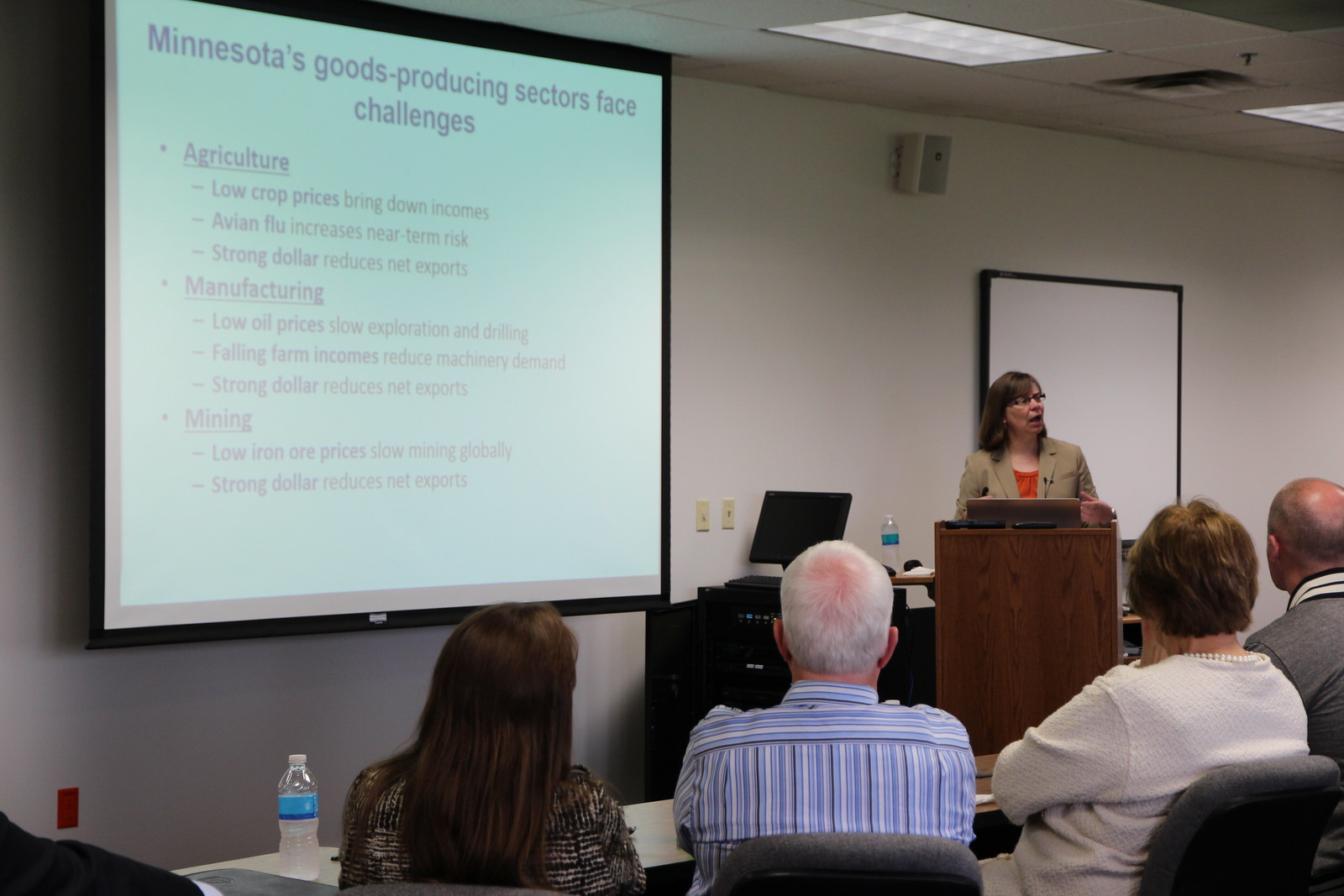In the image, a person is speaking at a brown wooden podium located in the middle-right section of the frame. The speaker, a woman, is addressing a classroom of attendees seated on white chairs with white tables in front of them. At least four individuals are prominently seated at the front table. 

On the far left side of the picture, a woman with long brown hair wears a brown sweater and has a water bottle placed in front of her. Next to her sits a man in a blue, white, and black pinstriped button-down shirt, with white hair. To his right is an individual with short hair, about neck-length, who is wearing a white sweater. Seated next to this person is another with a gray T-shirt; they have sparse, grayish hair, indicating balding.

The speaker is presenting a slideshow visible to her right (the viewer's left side). The slide's header reads, "Minnesota's Goods Producing Sectors Face Challenges." The presentation covers different categories, namely agriculture, manufacturing, and mining, with each category title underlined for emphasis.